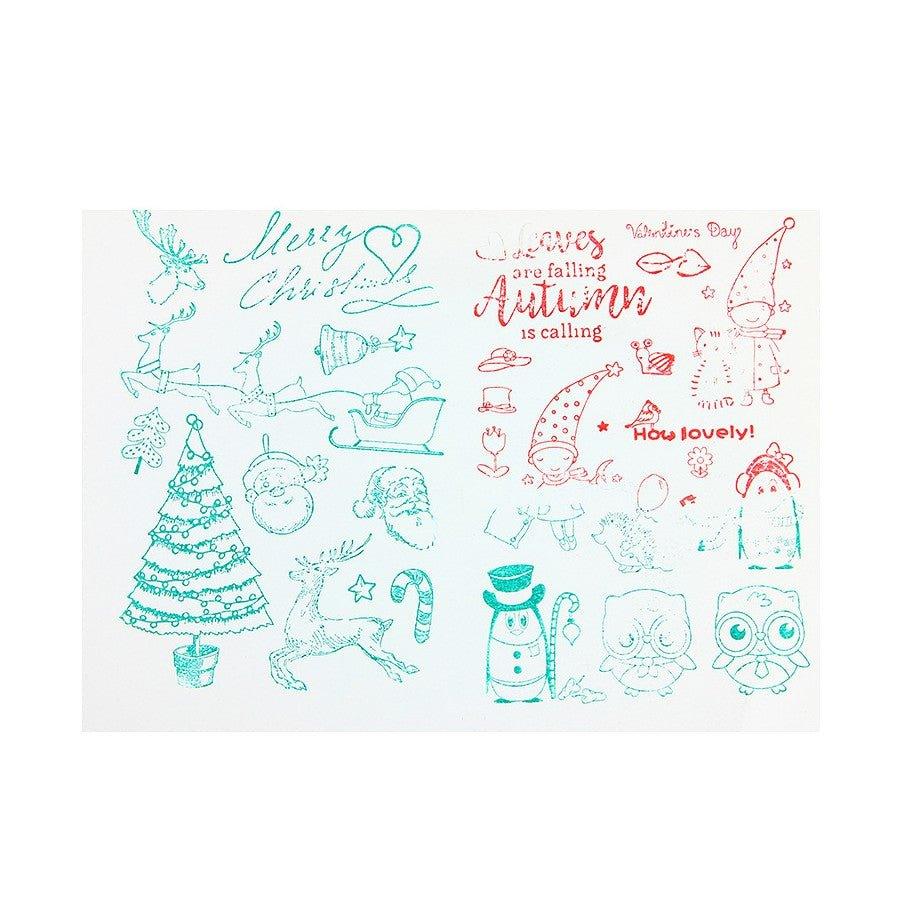This is an illustration on a white piece of paper, featuring a variety of holiday and seasonal stamps predominantly in green and red. On the left side, green Christmas-themed stamps include a reindeer, a "Merry Christmas" text with a heart, Santa Claus with his sleigh and two reindeer, a Christmas tree adorned with lights, and candy canes. There's also a green snowman holding a candy cane. Scattered among these are blue-colored stamps of owls with glasses and a penguin wearing a top hat, holding what looks like a fishing rod with an ornament on the end. On the top right section, red stamps feature autumn and Valentine's Day themes, including one with the text, "Leaves are falling, autumn is calling." This section also includes whimsical illustrations such as a little girl in a long pointed hat next to a cat, a flower, a vintage hat, and a snail. Mixing both red and green, there's a cute penguin with a bow on her hair and another little girl with a pointy hat and a star.